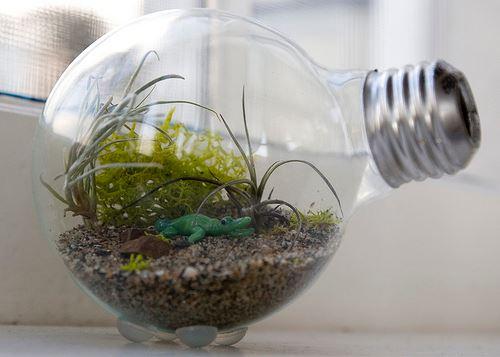The image showcases a cleverly crafted miniature terrarium housed inside a light bulb-shaped glass container that is laid on its side. The terrarium features a variety of miniature greenery, including green and brown grass, and possibly a Spanish moss-type air plant. Immersed in the soil, which occupies half of the round bulb, are bits of white rock. A tiny, fake green alligator is also nestled among the plants, adding a whimsical touch. The silver spiral at the end mimics the screw-in portion of a real light bulb, enhancing the illusion. To stabilize the bulb, it rests on four small, half-round glass feet that resemble decorative marbles. The scene appears against a predominantly white backdrop featuring a clear window and a countertop. The overall setting is bright with subtle accents, highlighting the terrarium’s intricate details and imaginative design.